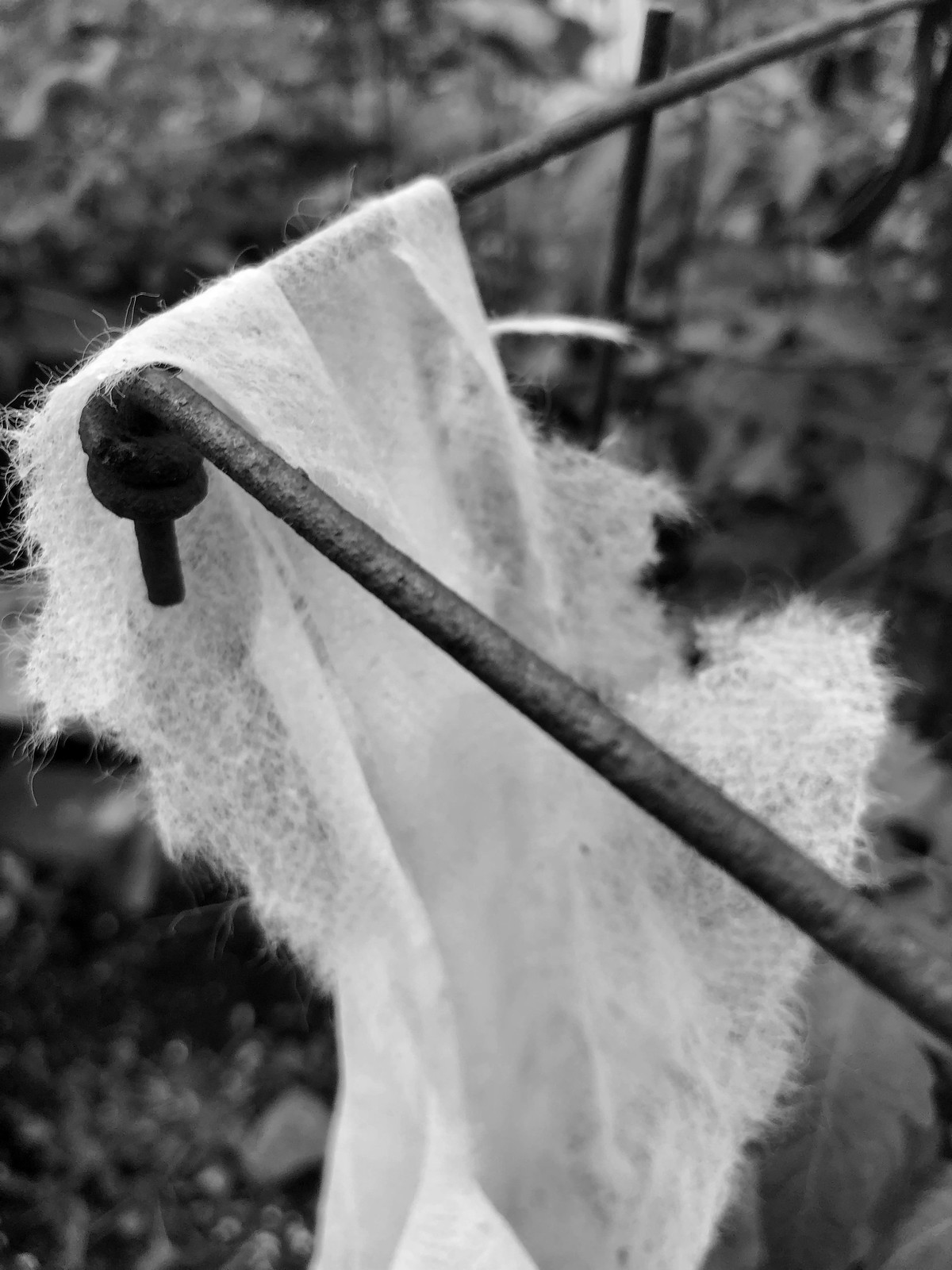This black and white photograph features a prominently frayed piece of white cloth or cotton, which is draped over a square-shaped metal rod structure composed of multiple rods. The fabric, appearing predominantly in the center of the image, hangs over one rod intersecting at an iron bar above it, which has a curved end with a large screw protruding from it. The background is blurred but showcases a natural outdoor setting with indistinct tree stems, leaves, dirt, and perhaps a few other plants. There are no people, names, dates, or locations identifiable in the photograph. The entire scene is rendered in shades of black, white, and gray, conveying a sense of minimalist simplicity within a natural environment.